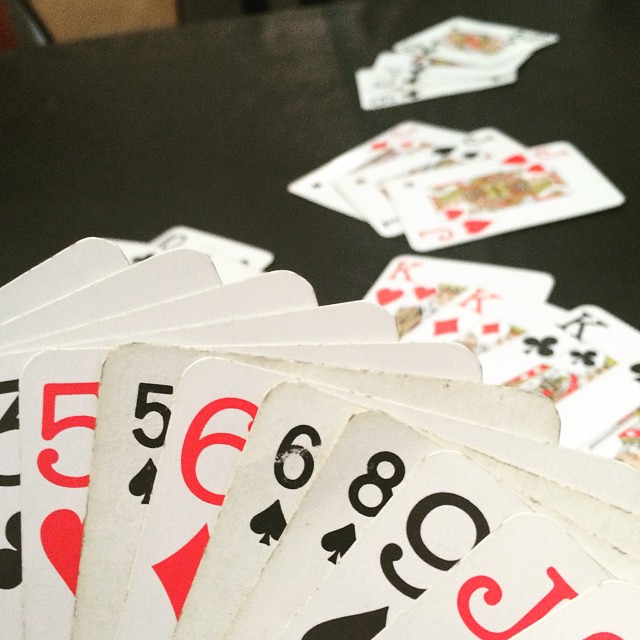A detailed close-up image showcases a fanned hand of standard playing cards held prominently in the foreground. The hand contains eight cards, listed sequentially from left to right: three of clubs, five of hearts, five of spades, six of diamonds, six of spades, eight of spades, nine of spades, and a partially obscured jack whose suit is not visible. 

In the background, a black playing card table displays multiple hands of cards arranged in various formations. Directly behind the main hand, a set of four kings is spread, three fully visible and a corner of the fourth peeking out. Above the kings, three jacks are laid out, and above them, another set of four cards is partially visible, including at least one queen. The table is cluttered with an assortment of cards, emphasizing the theme of a lively card game in session.